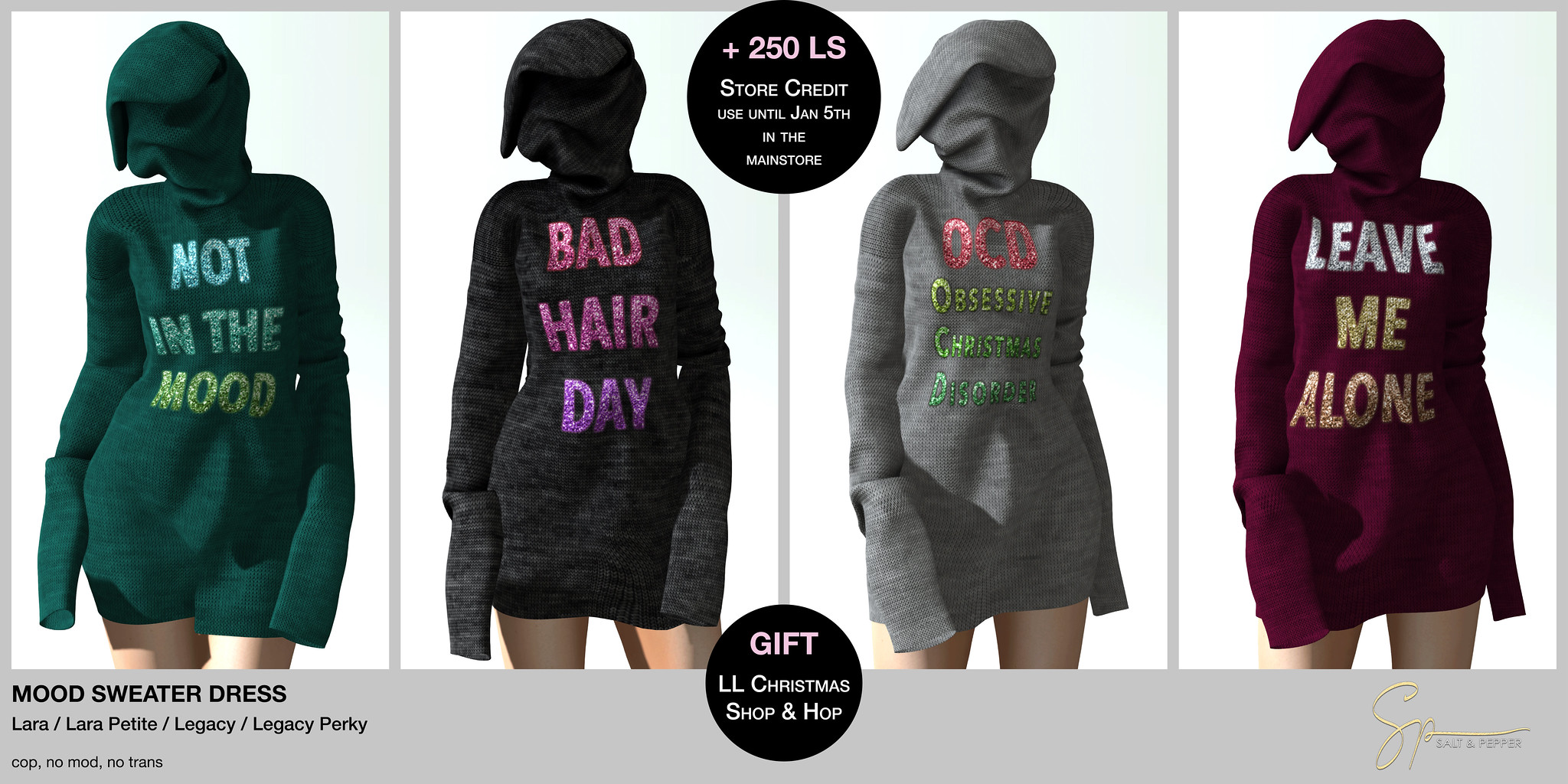This advertisement showcases a collection of one-piece sweater dresses that double as hoodies with full-face coverage. The dresses, resembling oversized hoodie-sweater hybrids, come in various colors: sea moss green, gray, dark black, and red. Each dress features playful and snarky word graphics, such as "Not in the Mood," "Bad Hair Day," "Obsessive Christmas Disorder (OCD)," and "Leave Me Alone." These messages stand out in glitter and metallic sheens, with "Leave Me Alone" stylishly depicted in silver and gold, and "Bad Hair Day" in purples and pinks. In the image, the models' faces are completely covered by the hoods, adding a unique twist that makes the dresses look like they can be worn backwards or as masks. Additionally, promotional text in the advertisement includes offers like "+250 L.S. store credit, use until January 5th in the main store" and highlights a "Gift, L.L. Christmas Shop and Hop," with a prominent "Mood Sweater Dress" caption at the bottom.